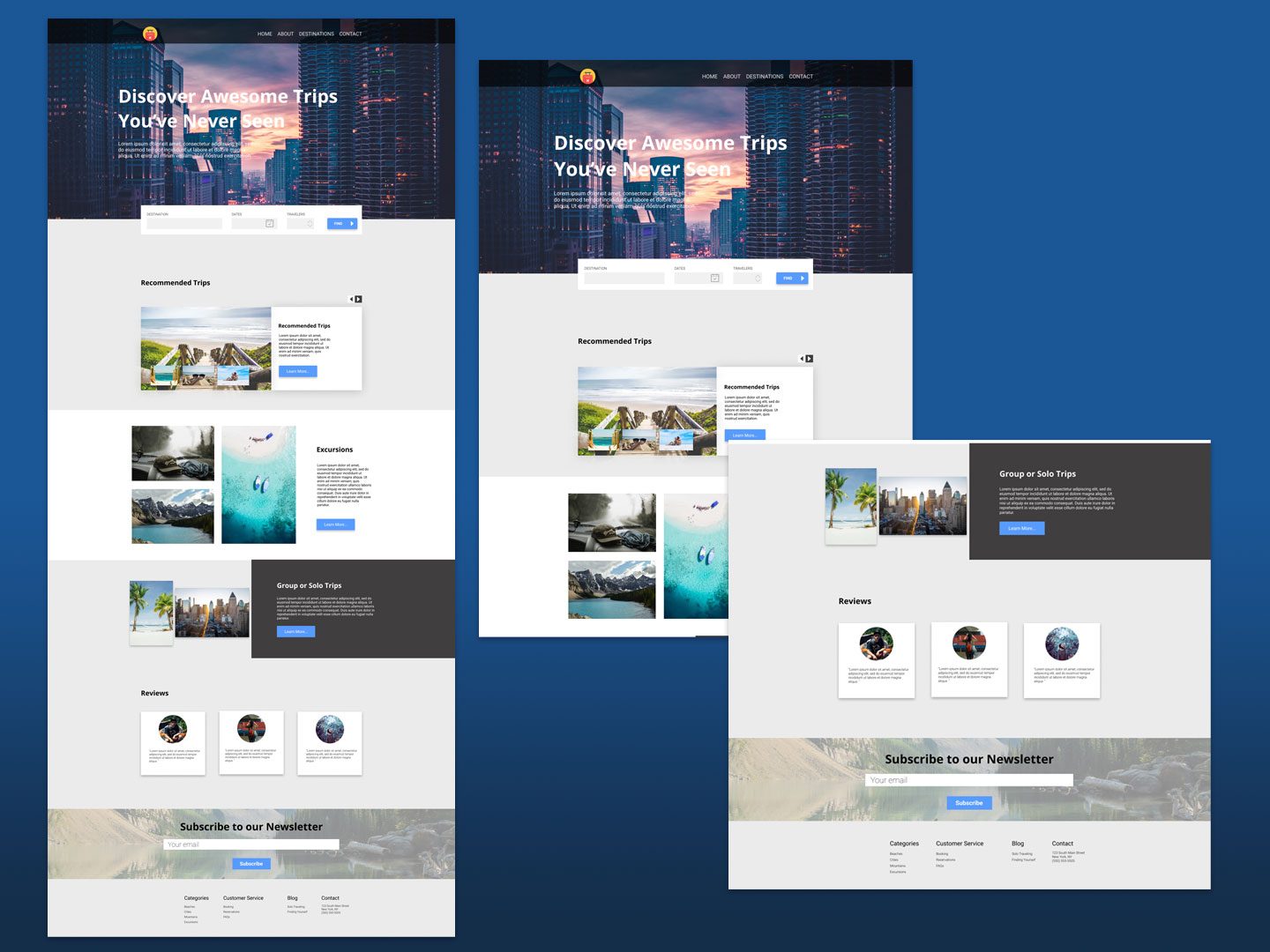The image is a composite of several screenshots of a website that promotes travel destinations. The leftmost section prominently features the tagline, "Discover awesome trips you've never seen." Below this tagline, although the text is too small to read, there appear to be example photos showcasing various travel destinations. Moving to the middle of the composite, this screenshot looks similar but presented in a smaller format, possibly a resized version or a mobile view. Lastly, the rightmost screenshot displays the bottom portion of the original left section, focusing on additional destination photos and providing a more comprehensive view of the website's layout dedicated to encouraging travel inspiration.